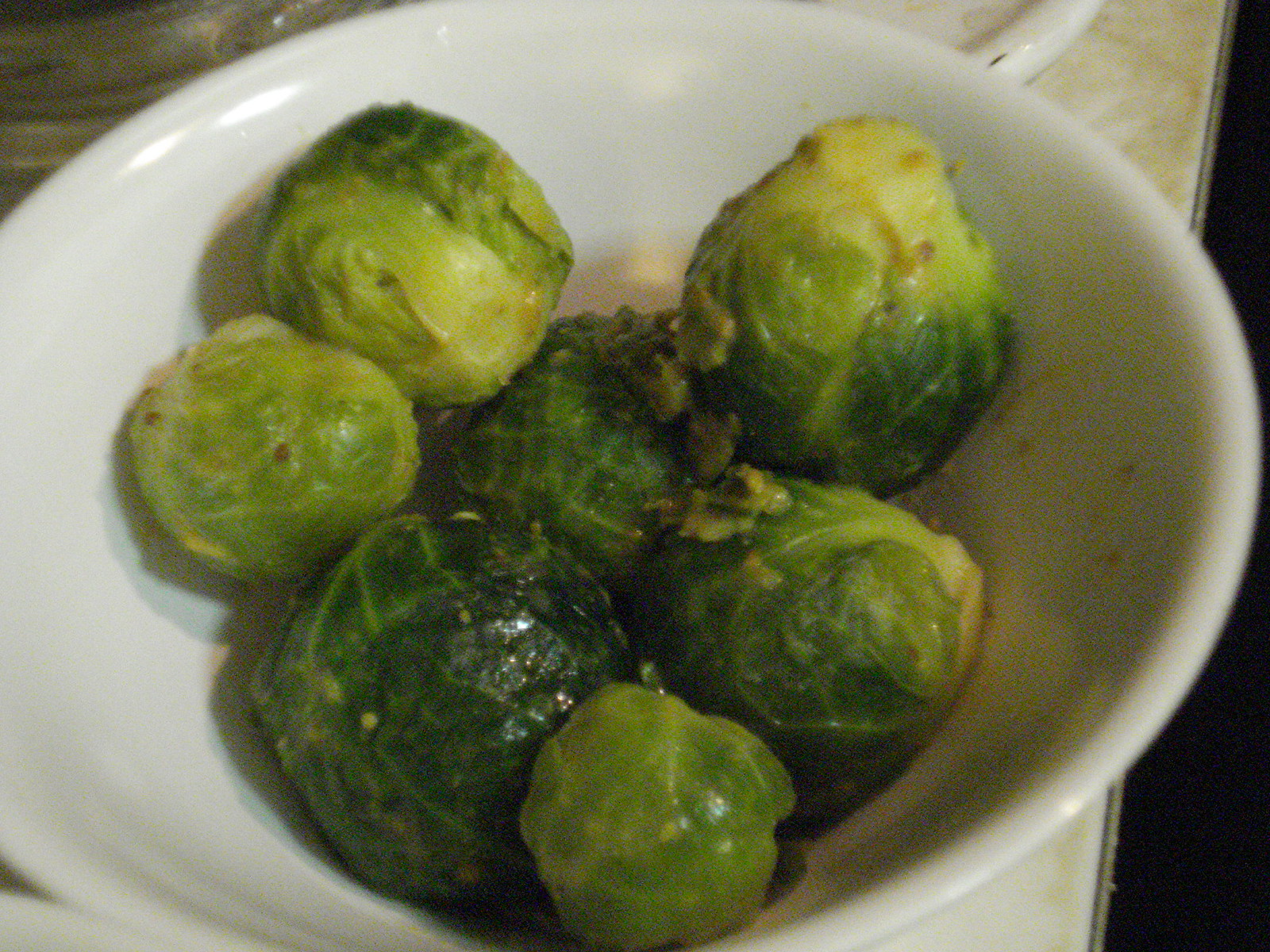This is a close-up photograph of a small white ceramic bowl containing seven cooked Brussel sprouts. The sprouts appear shiny, as if they were cooked in oil or butter, and are sprinkled with a seasoning that might be garlic or onion powder. There are a couple of large, vibrant green Brussel sprouts positioned at the bottom of the bowl, while the five smaller, more yellowish sprouts surround them. The bowl rests on what seems to be a white or cream-colored countertop with yellowish veining, possibly made of marble or granite. The image's low-light setting renders it grainy and adds a reflective quality to the Brussels sprouts, perhaps from the kitchen lighting. In the upper right corner, a vague white utensil is visible. Overall, the bowl and its contents are the focal point of the picture.